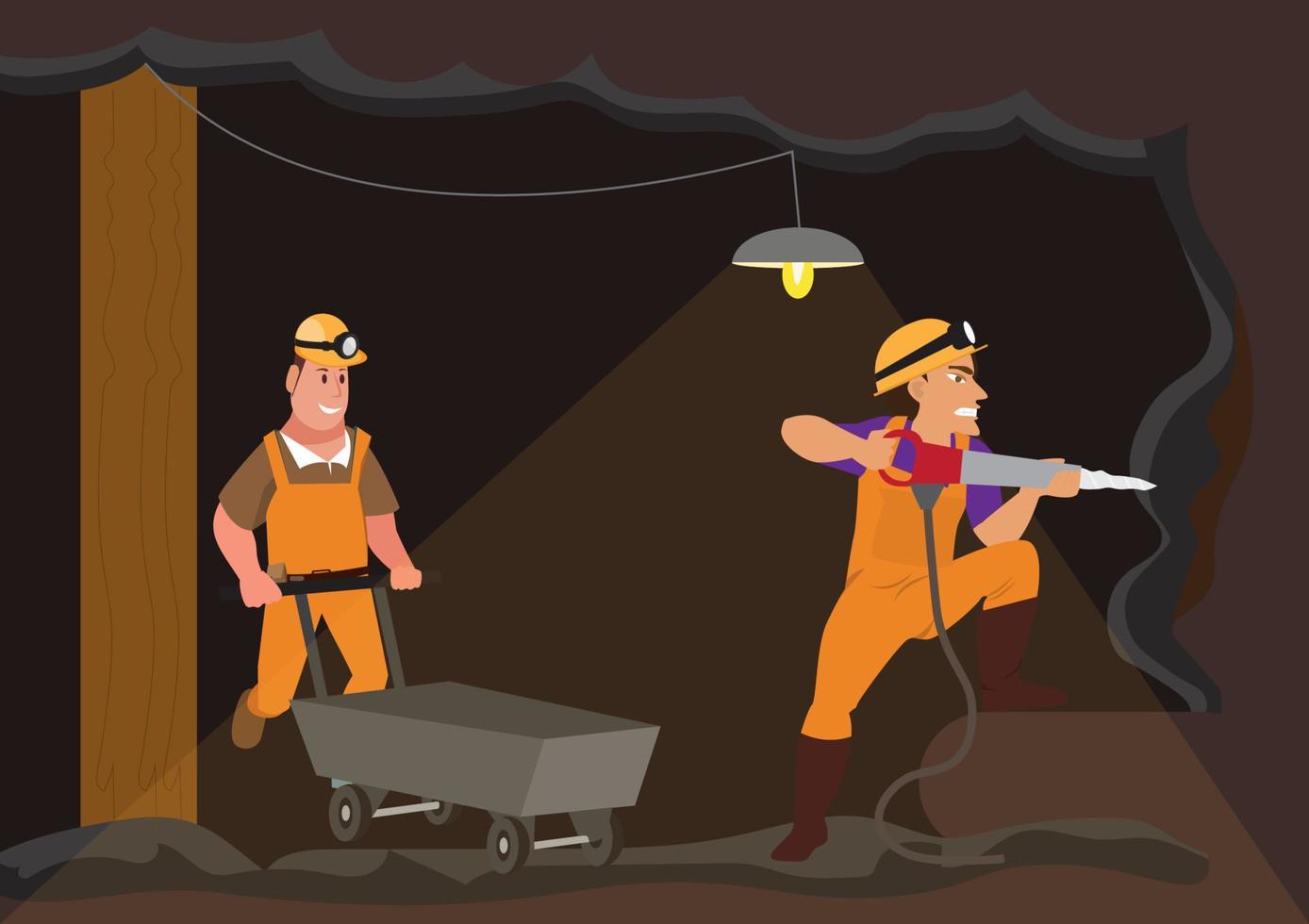This detailed illustration, either hand-drawn or computer-animated, depicts a cartoonish scene of two miners working in a small underground coal mine. The image shows a cutaway view of the mine, where the ground serves as the top and bottom borders. To the left, a wooden support beam holds up the ceiling, from which a light bulb lamp hangs on an electrical wire, illuminating the cave. 

On the right side, a miner with a darker complexion is seen wearing orange overalls, a purple shirt, and brown boots. He sports a hard hat with a headlight and is actively drilling into the cave wall with an electric or pneumatic drill, evident from the cord attached to the tool. His left leg is perched on a rock to give him leverage. 

Behind him, moving towards the right, is another miner who has white skin and wears similar orange overalls but with a brown shirt. He is pushing an empty four-wheeled wheelbarrow, more akin to a trolley car with a handle. He is smiling and appears ready to collect the debris from the drilling operation to transport it away. Scattered rocks decorate the bottom of the mine, completing this dynamic and industrious scene.